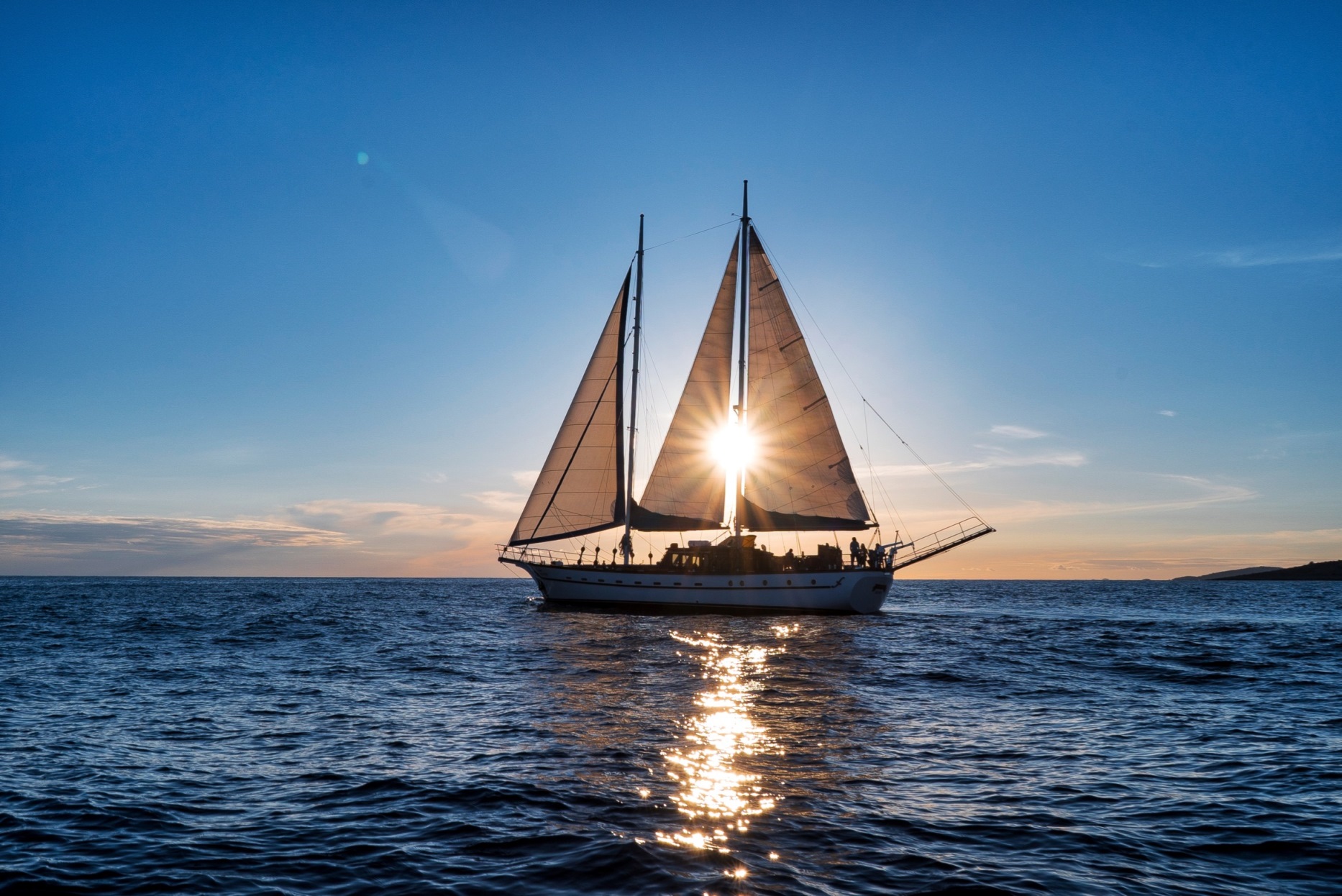In this stunning photograph taken either shortly after sunrise or before sunset, a sailboat stands majestically at the center of the frame, bathed in a golden, peachy light. The sky, a vibrant blue with a peach-colored hue near the horizon, is adorned with a few scattered clouds. The sun, positioned behind the sailboat's three cream-colored, triangular sails, shines brilliantly, casting light through the sails and illuminating the scene with an elegant glow. The calm, rich blue ocean below mirrors this radiant sunlight, creating a beautiful reflection. Several people are seen standing on the deck of the white sailboat, likely tourists enjoying a serene maritime experience. Towards the right side of the photograph, the outline of distant mountains provides a scenic backdrop, enhancing the overall tranquility and beauty of the scene.